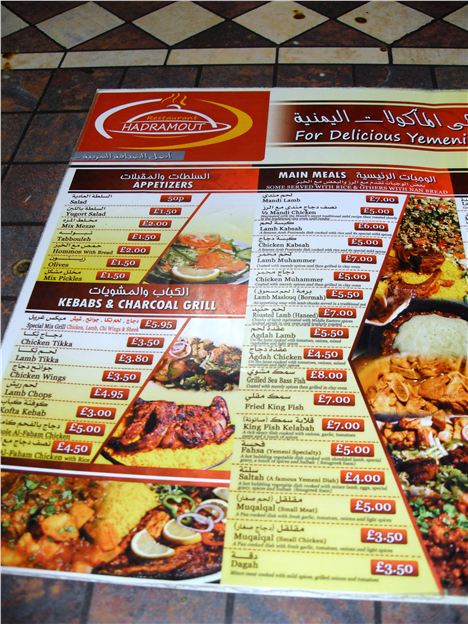The image is a close-up of a vibrant and visually appealing takeaway menu from Hadramout Restaurant, prominently featuring the phrase "Four Delicious Yemeni" at the top. The menu, which lies on a slightly dirty restaurant floor with visible food stains, is printed on a yellow sheet with red text, making the details pop against the background. It is organized into sections for appetizers, kebabs and charcoal grill, and main meals. The appetizers listed include salad with lettuce, lemon wedges, and cucumbers; hummus and bread; and a mixed pickle dish. The kebabs and charcoal grill section offers chicken tikka, lamb tikka, chicken wings, and lamb chops. For the main courses, diners can choose from dishes like lamb mahammer, chicken mahammer, Agdala lamb, Agdala chicken, grilled sea bass fish, Kingfish kebab, Fasa, Salta, and Daga. The prices, marked with the pound symbol, suggest the restaurant is located in the UK. Adding to the menu's allure are stunning visual images of the food, including plates of salad, grilled meats with lemon wedges, red onions, and green bell peppers, and chicken wings.